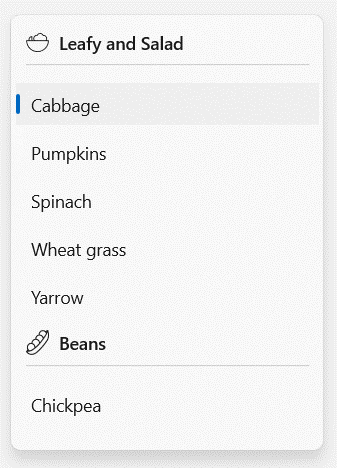The image features a screenshot with a gray background. Central to the image is a white box containing a picture of a bowl, which appears to be filled with a salad made up of leafy greens and possibly other vegetables. The top of the white box prominently displays the word "leafy" in bold text, followed by the word "salad." Below the salad image, a list of items is presented, each item accompanied by a small icon and text.

The list includes:

1. **Cabbage** - Marked by a blue line to its left.
2. **Pumpkins** - Listed as the next item.
3. **Spinach** - Appearing third in the sequence.
4. **Wheatgrass** - Listed fourth.
5. **Yarrow** - Featured fifth.
6. **Beans** - Bolded text with an accompanying image of a bean pod containing four beans.

A thin, light gray line separates this part from the next item:

7. **Chickpea** - The final item on the list.

This arrangement highlights various vegetables and legumes, probably suggesting their use in preparing the salad depicted in the central image.